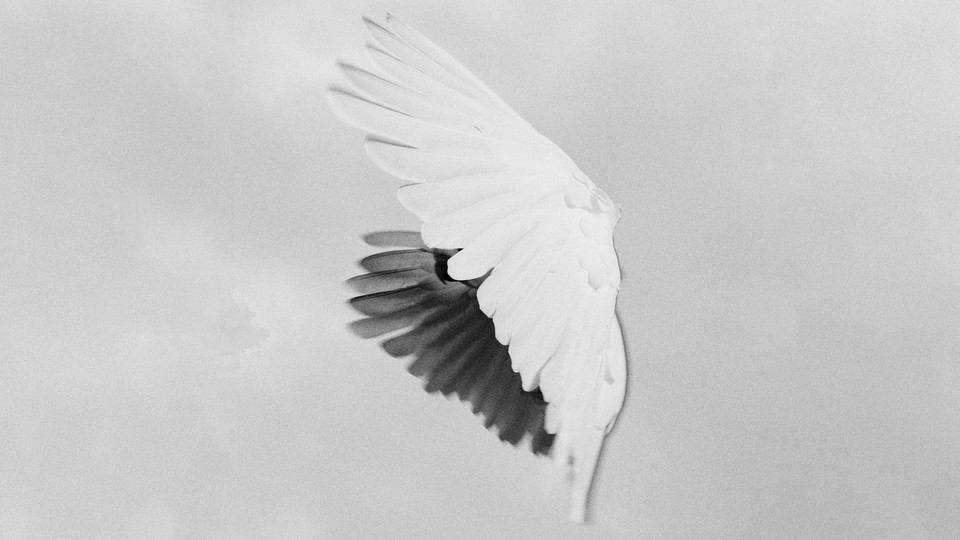The image showcases a detailed artistic depiction of a bird with a focus on its wing and a corresponding shadow. Centered in the composition, the bright white wing, which appears to be large and majestic, is subtly tilted to the left. Directly beneath and to the left, positioned almost as if mirroring the wing above, is its shadow—rendered in a blackish-gray hue. The entire scene is set against a plain gray background, emphasizing the contrast between the wing and its shadow. The artwork could be a watercolor, oil painting, or digital piece, emphasizing the graceful motion of the bird with its distinct white and black feathers. Notably, there is no text within the image. The overall style suggests a careful and artistic study of the bird's flight, captured in a minimalist yet striking visual manner.